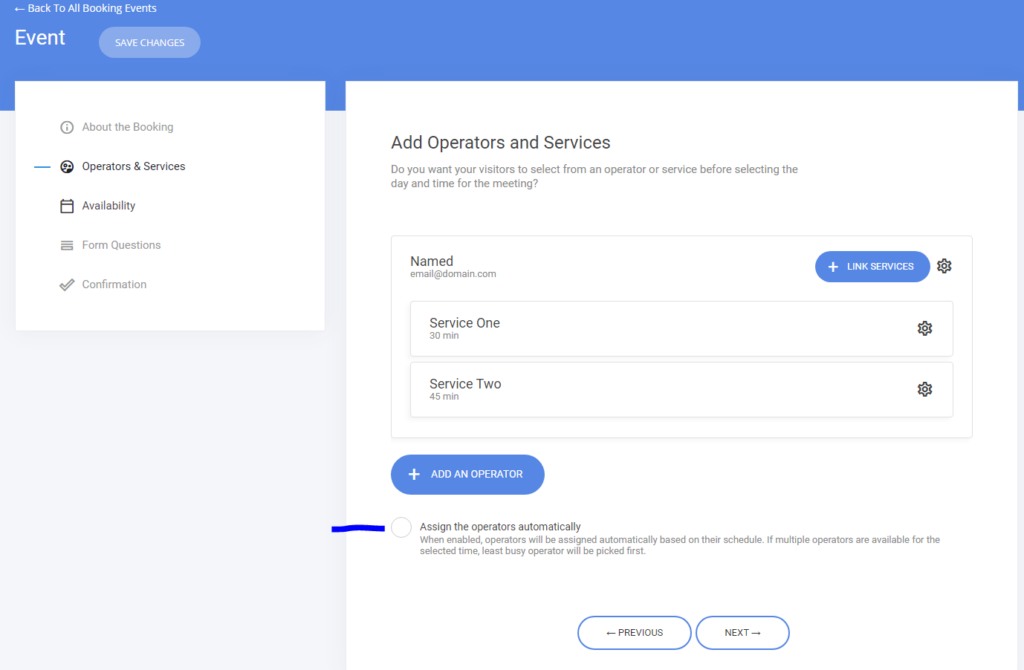The image depicts an interface with a blue border at the top, featuring a button labeled "Back to All Booking Events". Beneath this button is another button titled "Save Changes". Below these, on the left side, there is a list displayed in a white square containing items such as "About the Booking", "Operation of Services", "Availability", "Form Questions", and "Confirmation". Each of these items is accompanied by an icon to its left that visually represents its category. 

To the right of this list is a larger white square that prompts users to "Add Operators and Services." Below this prompt, the text asks, "Do you want your visitor to select from an operator or service before selecting the day and time for a meeting?" Following this question is a series of input fields labeled "Name", "Service One", and "Service Two". Below these fields, there is a blue box with the text "+ Add an Operator". At the bottom of the interface, there are two buttons labeled "Previous" and "Next" for navigation purposes.